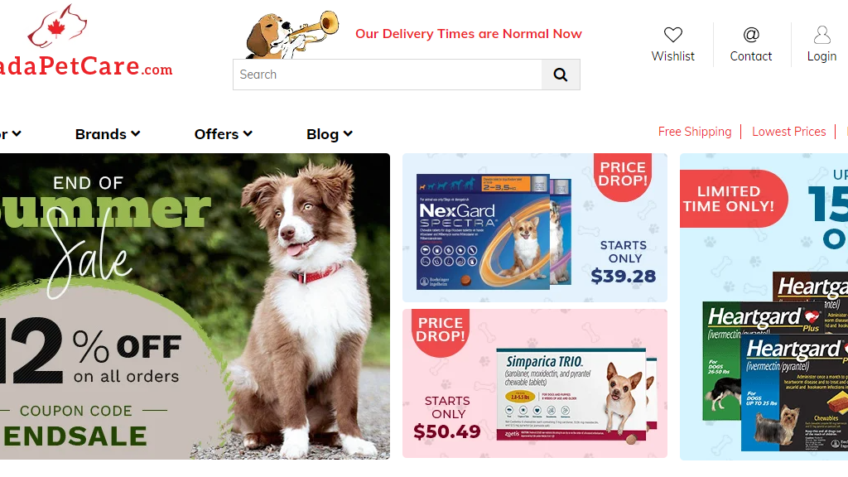This screenshot captures a vibrant and detailed image of a pet care website, DAPetCare.com. At the top left corner, there's a partially visible logo featuring a dog's head and the website name. Dominating the upper center is a whimsical image of a brown and white dog playing a trumpet with a message stating, "Our delivery times are normal now." Beneath this playful visual is a conspicuous search bar.

The bottom portion is a bustling display of ads showcasing various pet care products. To the left, an ad announces an "End of Summer Sale," offering a 12% discount on all orders with a mention of a coupon code. The background featuring this ad is lush with green trees and bushes, adding a refreshing natural feel. Adjacent to it, a cheerful brown and white dog sporting a red collar playfully sticks his tongue out, looking happily to the left.

In the middle of the layout are two vertically stacked rectangular ads. The top rectangle, with a blue background, features a brown and white dog promoting "NextGuard" with a price drop starting at $39.28. The lower rectangle, adorned in pink, advertises "Parika Trio" flea and tick medicine with an image of a chihuahua, listing a starting price of $50.49.

On the far right, another ad with a light blue background promotes "HeartGuard," featuring three boxes of the heartworm medication decorated with dog images. The ad hints at a limited-time offer, though partially cut off on the right side.

Overall, the relevant details and colorful ads blend seamlessly, presenting a visually engaging and informative snapshot of all essential pet care deals and updates.